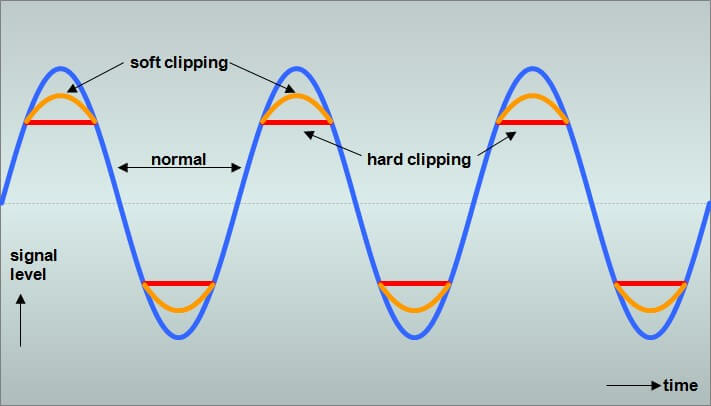The image is a detailed line graph depicting signal variations over time on a gray background. At the top of the graph, the term "soft clipping" is indicated, and beneath it, the word "normal" is placed with arrows pointing left and right. On the right side of the graph, the term "hard clipping" is accompanied by similar bidirectional arrows. The main feature of the graph is a royal blue wave-like curve that oscillates up and down, representing the signal levels over time. Within each wave, there is a soft, curved, gold line that aligns closely with the blue curve, indicating instances of soft clipping. Additionally, there are straight red lines cutting across the blue waves, marking instances of hard clipping. The overall layout suggests this is potentially a slide from a technical presentation highlighting the differences and effects of soft and hard clipping on signal quality.